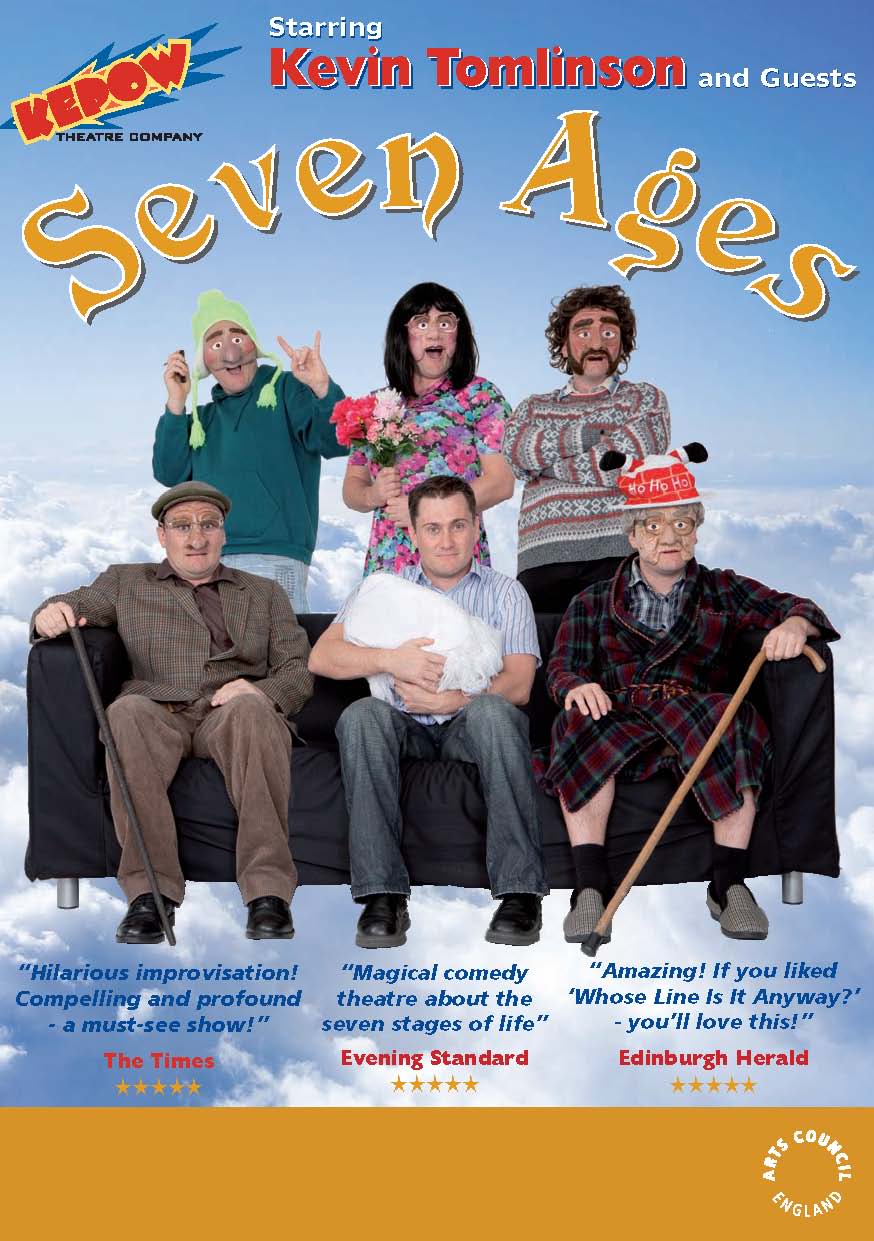This image is an advertisement for a comedy movie titled "Seven Ages" by the Kapow Theatre Company, prominently displayed in the upper section of the poster with curved yellow text. The poster features a group of six people arranged in two rows—three sitting on a sofa and three standing behind it—each wearing masks or costumes that contribute to a humorous appearance. 

Starting from the front row, two elderly-looking individuals sit on either end of the sofa, both holding canes and wearing masks that make them appear very old. The man in the middle, the most regular-looking person among them, is holding a baby in a blanket. In the back row, the three standing individuals are also in masks, but these are unlike the elderly masks worn by those sitting. One person is in a green beanie, another, a woman in a dress holding flowers, and the last has somewhat bizarre features including facial hair and is wearing a sweater or a winter hat.

Additionally, the upper left corner of the poster features red and white text that reads "Kapow" and "starring Kevin Tomlinson and guests." The bottom section of the poster includes various blue quotes lauding the movie's comedic impact and performances, with red text providing the sources of these accolades. These reviews are complemented by orange stars representing five-star ratings. At the very bottom in an orange bar, white text inside a circle marks the involvement of Arts Council England. This vibrant and detailed advertisement hints that the movie delivers a hilarious improvisational experience similar to shows like "Whose Line is it Anyway?" and is likely targeted at a British or Scottish audience.